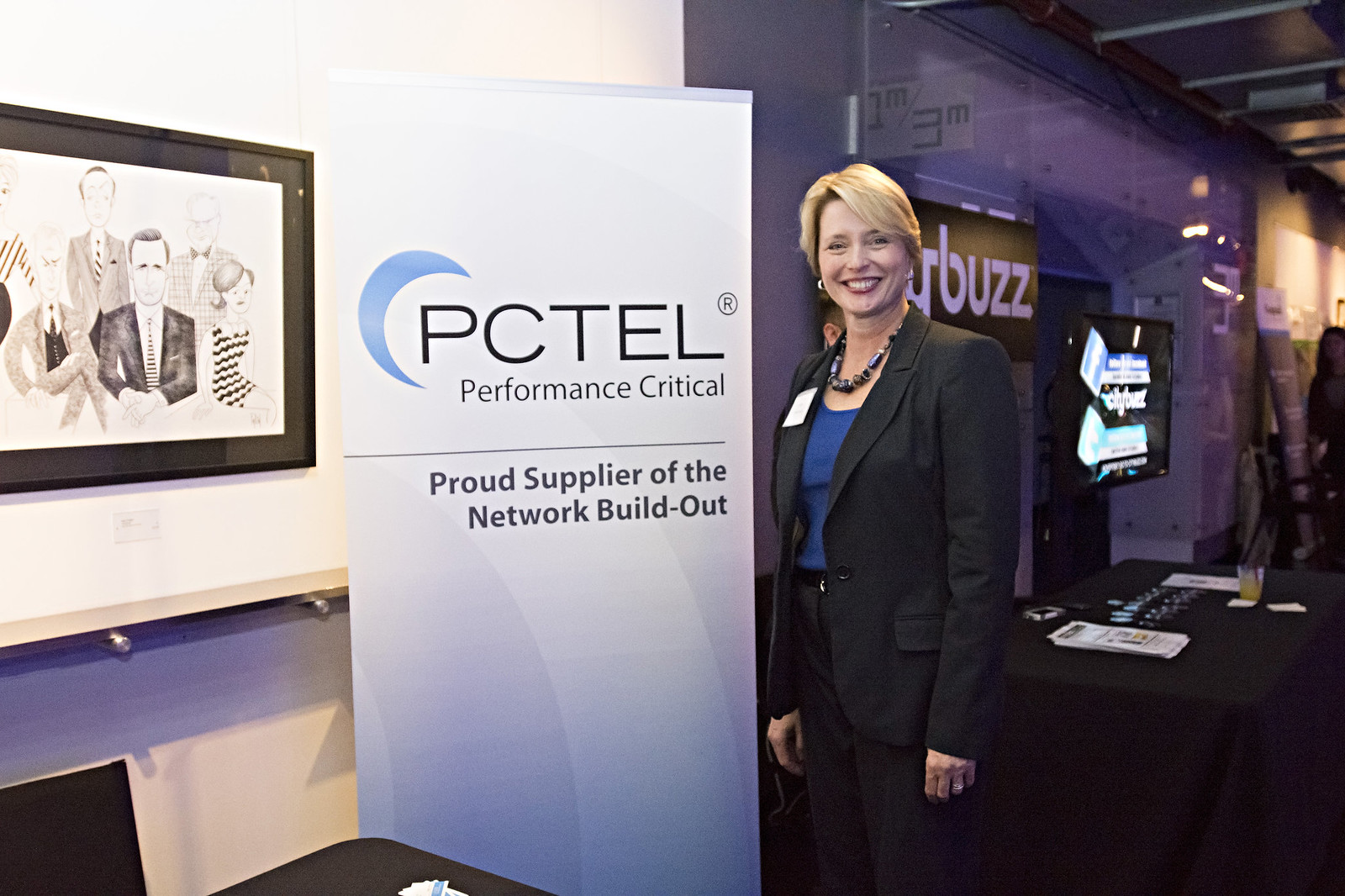In the photograph, a smiling white woman with short blonde hair poses next to a tall, rectangular standing banner situated to her left. The woman, standing slightly to the right, is wearing a black business coat over a dark blue blouse, black dress pants, and silver hoop earrings. She accessorizes with a beaded necklace featuring dark blue, black, and possibly brown jewels, as well as a ring on her left ring finger. Her hands rest at her sides against a background of a white-painted wall.

The banner she poses beside has a white background with blue radial stripes at the center. At the top of the banner, in black text, are the words "PCTEL Performance Critical." Just below that, the text reads, "Proud supplier of the network build-out." To the top left of the text is a blue crescent shape. 

In the background, to the left of the banner, there is a framed image depicting a caricature of five people, though glare from the lighting makes it difficult to distinguish details clearly. To the right of the woman, there is a black table covered with various flyers and other items. Above the table, there's a TV mounted on a stand with two visible logos, and above that is another signboard. In the far right background, there is a partially visible person, slightly cut off by the frame.